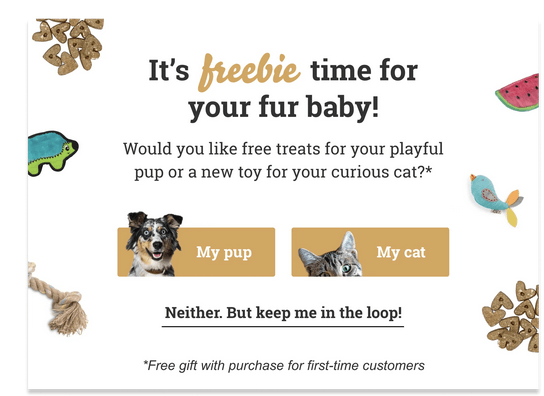This image, set against a white background, features a detailed screenshot framed by a thin gray line on the left and right, and a thicker gray line running horizontally along the bottom. In the upper-left corner, there is an illustration of heart-shaped brown dog cookies. Below this, a porcupine depicted in blue and green colors is showcased, followed by a rope bone toy in the lower left corner.

On the upper right side, there is a colorful illustration of a watermelon slice, beneath which a bluebird illustration is placed. Additional heart-shaped brown dog cookies are also visible in this area. 

Centrally, at the top, bold black text reads, "It's freebie time for your fur baby," with the word "freebie" highlighted in light brown text. Below this message are two interactive buttons: one on the left labeled "My Pup," featuring an image of a Border Collie, and another on the right labeled "My Cat," displaying the face of a Tabby cat.

Towards the bottom, bold text offers a third option, "Neither, but keep me in the loop," with an underline emphasizing this phrase.